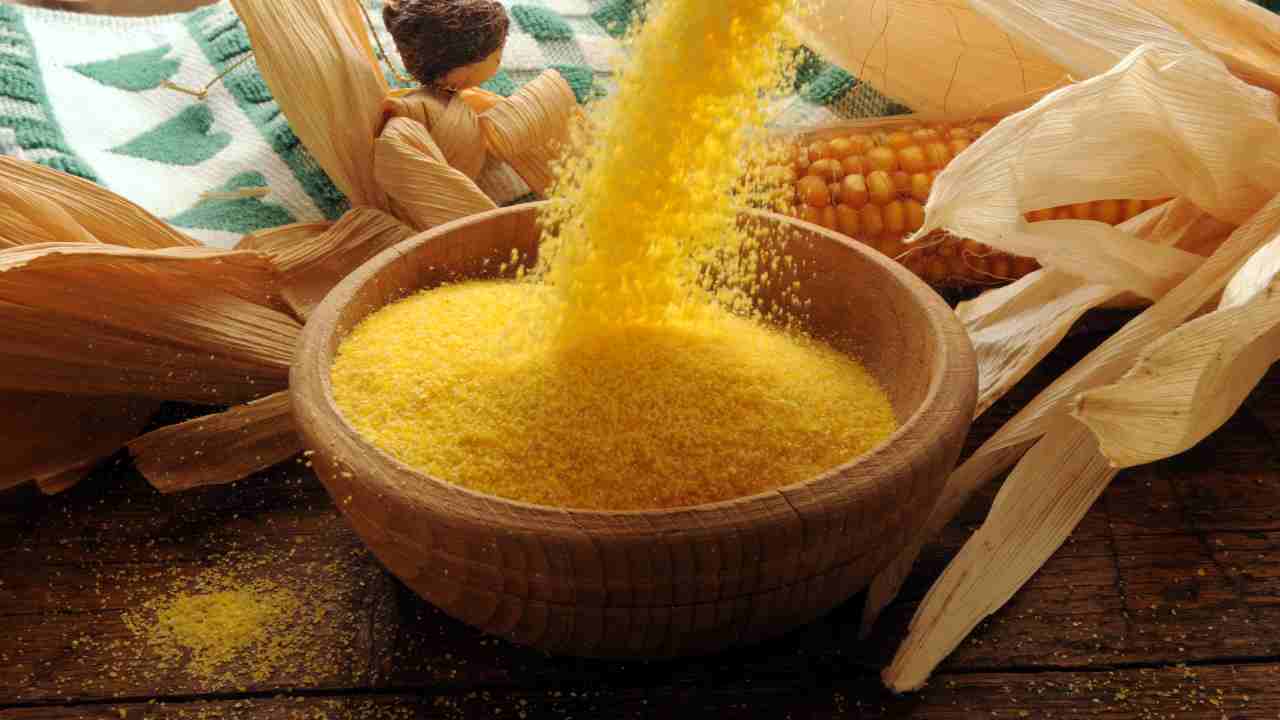In this image, a nearly full wooden bowl filled with fine yellow cornmeal grains is prominently displayed on a dark brown wooden table, resembling a picnic table surface. The cornmeal is being poured into the bowl from the top of the frame, with some grains visibly suspended in mid-air. Surrounding the bowl, there's a partially peeled ear of corn showcasing its yellow kernels and tan husk on the right side. Additional light tan corn husks are scattered to the left. In the background, at the upper left corner, a green and white towel featuring a heart pattern adds a touch of contrast to the rustic scene. All this, set on the rich wooden table, evokes a setting of active food preparation or cooking.